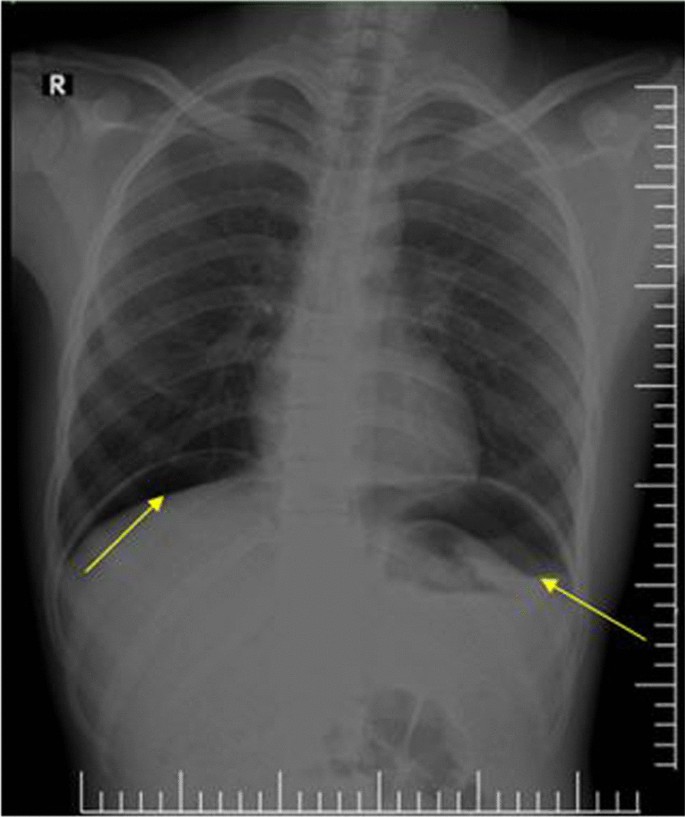The image is an x-ray of a person's chest, clearly displaying their ribcage and lungs against a black background. Both the left and right lungs are visible, with notable differences in their appearance; the right lung appears worse and is slightly larger, extending approximately one rib bone length more than the left lung. The left lung, in contrast, lacks significant curves and appears thick. The image also includes measuring lines: vertical lines on the right side resembling a ruler, and horizontal lines at the bottom positioned similarly, both devoid of numbers. Yellow arrows are present, with one located at the bottom right edge of the right lung, pointing upwards from the second short line on the vertical scale, and another arrow slightly higher on the left side pointing to a different area of the lung. The top left corner of the image features a white "R" encased in a black circle, indicating the right side of the x-ray.